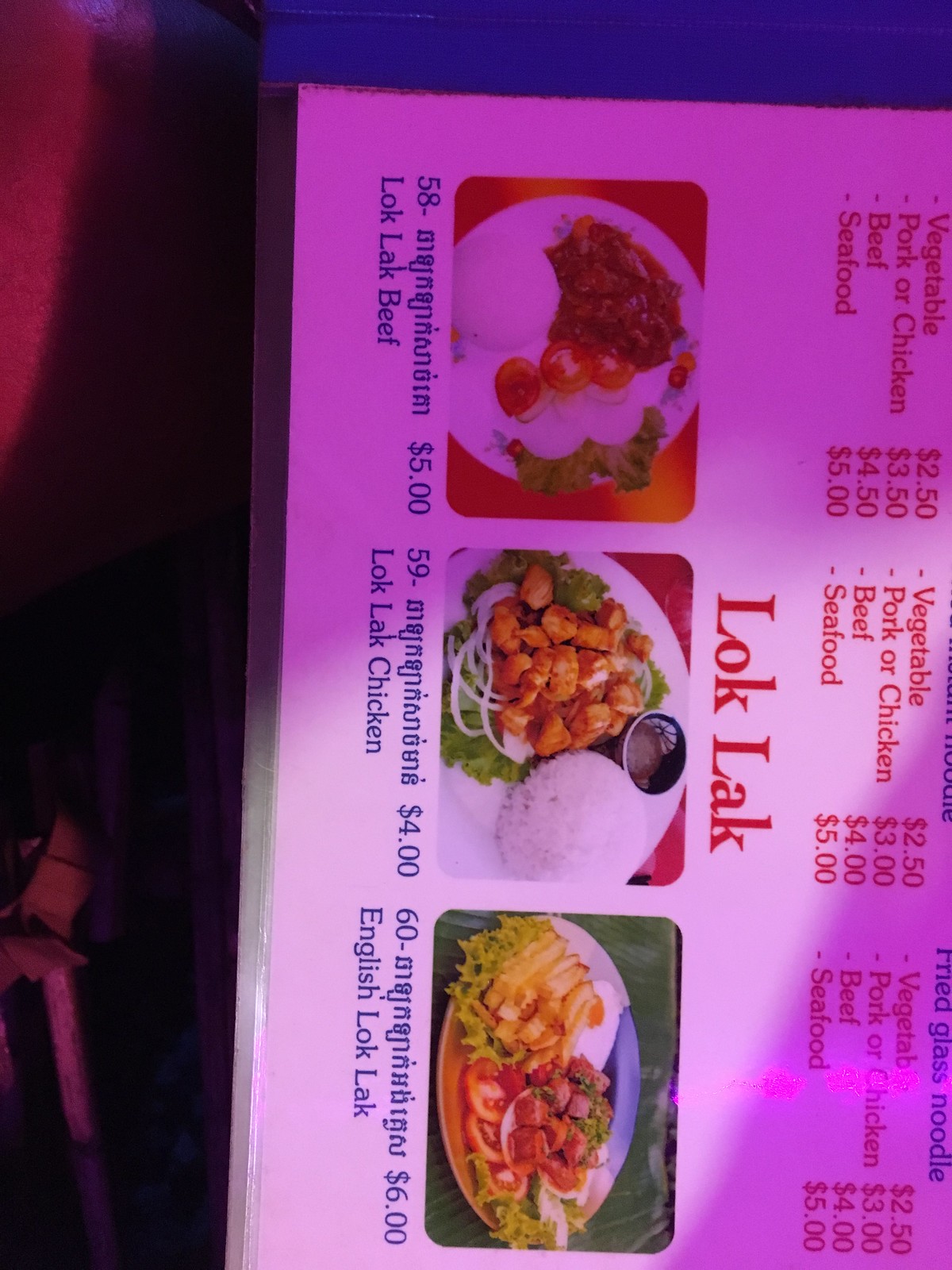This image depicts a food menu that needs to be rotated 90 degrees to the left to be viewed correctly. The photograph is slightly cut off, showing only two main sections of the menu. The lighting is dark with a bluish-purple hue cast over the menu, adding a vibrant but moody contrast to the visual.

The menu features multiple rows likely dedicated to various noodle dishes sectioned into three categories. Due to the cut-off, the type of noodle for the first column is unclear. However, it lists the following options and prices: vegetables ($2.50), pork ($3), beef ($4), and seafood ($5). 

The top of the next section hints at another noodle type, likely starting with the word "noodle," followed by the repeated price structure: vegetables ($2.50), pork or chicken ($3), beef ($4), and seafood ($5). The last visible column is labeled "fried glass noodles" in blue font. This section also displays the same price structure in red font: vegetables ($2.50), pork or chicken ($3), beef ($4), and seafood ($5).

At the bottom of this column, centered in large red letters, the word "Loklak" is displayed alongside pictures of the dishes. Menu item number 58 is Loklak beef priced at $5. Menu item number 59 features Loklak chicken for $4, and menu item number 60, referred to as English Loklak, is priced at $6.